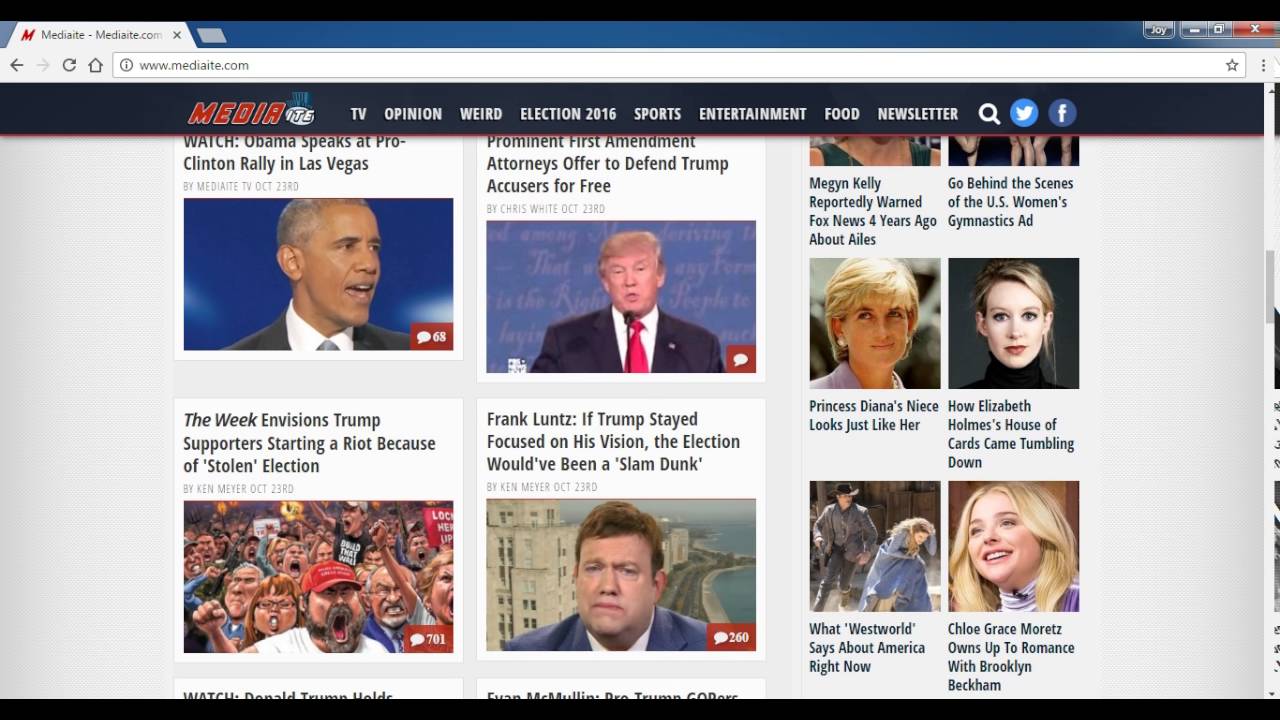Here is your cleaned-up and detailed caption for the described image:

---

A screenshot from the website Mediaite, featuring its distinctive file folder tab design on the top left. The URL shown is www.mediaite.com, with a star icon for adding the page to your favorites. The website's logo includes "Media" in red italicized letters while "ite" is set against an oval background.

A horizontal black navigation bar houses categories in white letters: TV, Opinion, Weird, Election 2016, Sports, Entertainment, Food, and Newsletter. To the right of these categories is a white search icon, followed by the Twitter bird and Facebook icons.

The main section of the screenshot displays several large photos and headlines on the left, with smaller thumbnail images and corresponding headlines on the right. 

**Left Column:**
1. **Top Left:** "Watch Obama Speaks at Pro Clinton Rally in Las Vegas" - features a large photo of President Obama and a red comment icon indicating the number of comments.
2. **Top Right:** "Prominent First Amendment Attorneys Offer to Defend Trump Accusers for Free" - features a large photo of Donald Trump with a comment icon.
3. **Bottom Left:** "The Week envisions Trump supporters starting a riot because of 'stolen election'" - includes a color editorial cartoon of Trump supporters wearing MAGA hats.
4. **Bottom Right:** "Frank Luntz: If Trump stayed focused on his vision the election would have been a 'slam dunk'" - showcases a photo of Frank Luntz with a shoreline and large building in the background.

**Right Column Thumbnails:**
1. "Megan Kelly reportedly warned Fox News four years ago about Ailes" - image of Megan Kelly.
2. "Go behind the scenes of the US Women's Gymnastics" - descriptive text cut off.
3. "Princess Diana's niece looks just like her" - image of the late Princess Diana.
4. "How Elizabeth Holmes's house of cards came tumbling down" - photo of Elizabeth Holmes pre-incarceration.
5. "What Westworld says about America right now" - still shot from the show Westworld.
6. "Chloe Graetz Moretz owns up to romance with Brooklyn Beckham" - photo of the actress Chloe Graetz Moretz.